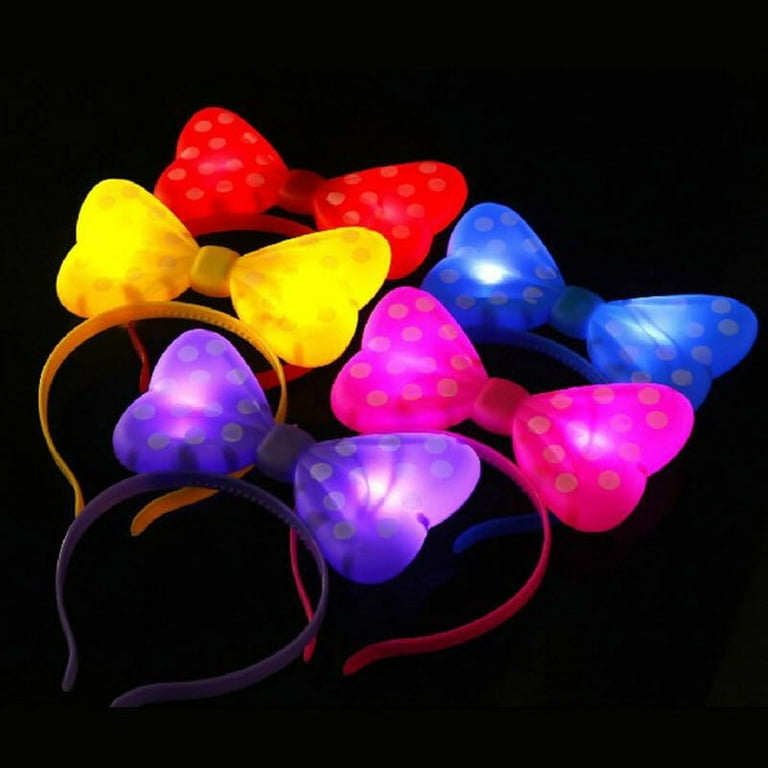The image portrays an online shopping product photo featuring a set of five colorful plastic headbands designed to resemble Minnie Mouse-style bows. The headbands are neatly stacked against a completely black background, each adorned with a large, translucent bow that lights up in bright neon colors. The bows are arranged in layers, with the light purple bow at the bottom, followed by a yellow bow, a pink bow, a red bow, and a blue bow, all cascading towards the left lower corner. Each bow, with its heart-shaped loop, adds a whimsical touch, reminiscent of children's accessories likely found in theme parks like Disneyland. The bows are decorated with light gray polka dots, with the yellow one featuring slightly darker yellow dots, enhancing the playful and festive appearance of these illuminated headbands.